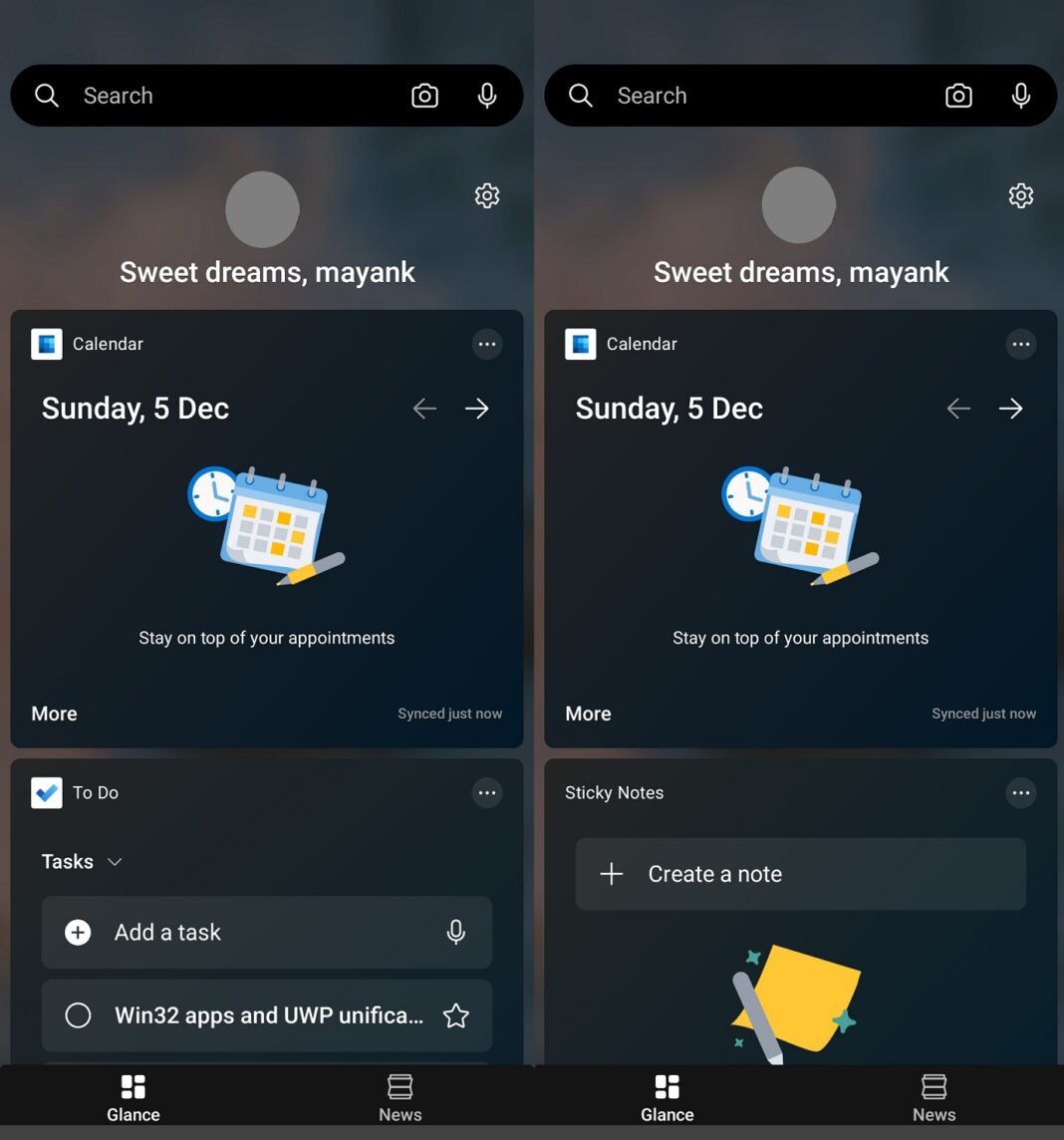The image depicts two cell phone screenshots placed side by side. Across the entire bottom of the image is a black bar which suggests that this is a composite screenshot of the two original screenshots. Within this black bar, four segments contain the words "glance," "news," "glance," and "news" respectively, each accompanied by distinct icons relevant to their titles. 

The primary background color of the screenshots is a blend of black and gray. The left screenshot is a mirror image of the right one, with minor deviations near the bottom. At the top, both screenshots feature a search bar equipped with icons for search, camera, and microphone functionalities. The phrase "Sweet Dreams MyMec" is prominently displayed near the top on both sides, accompanied by a circular image placeholder for a profile picture and a settings icon positioned to the right.

Beneath this section, both screenshots indicate the calendar date "Sunday, December 5th," with a calendar icon centrally placed. The primary difference between the two screenshots lies near the bottom: the left screenshot includes a section labeled "To-Do," while the right screenshot features a section labeled "Sticky Notes."